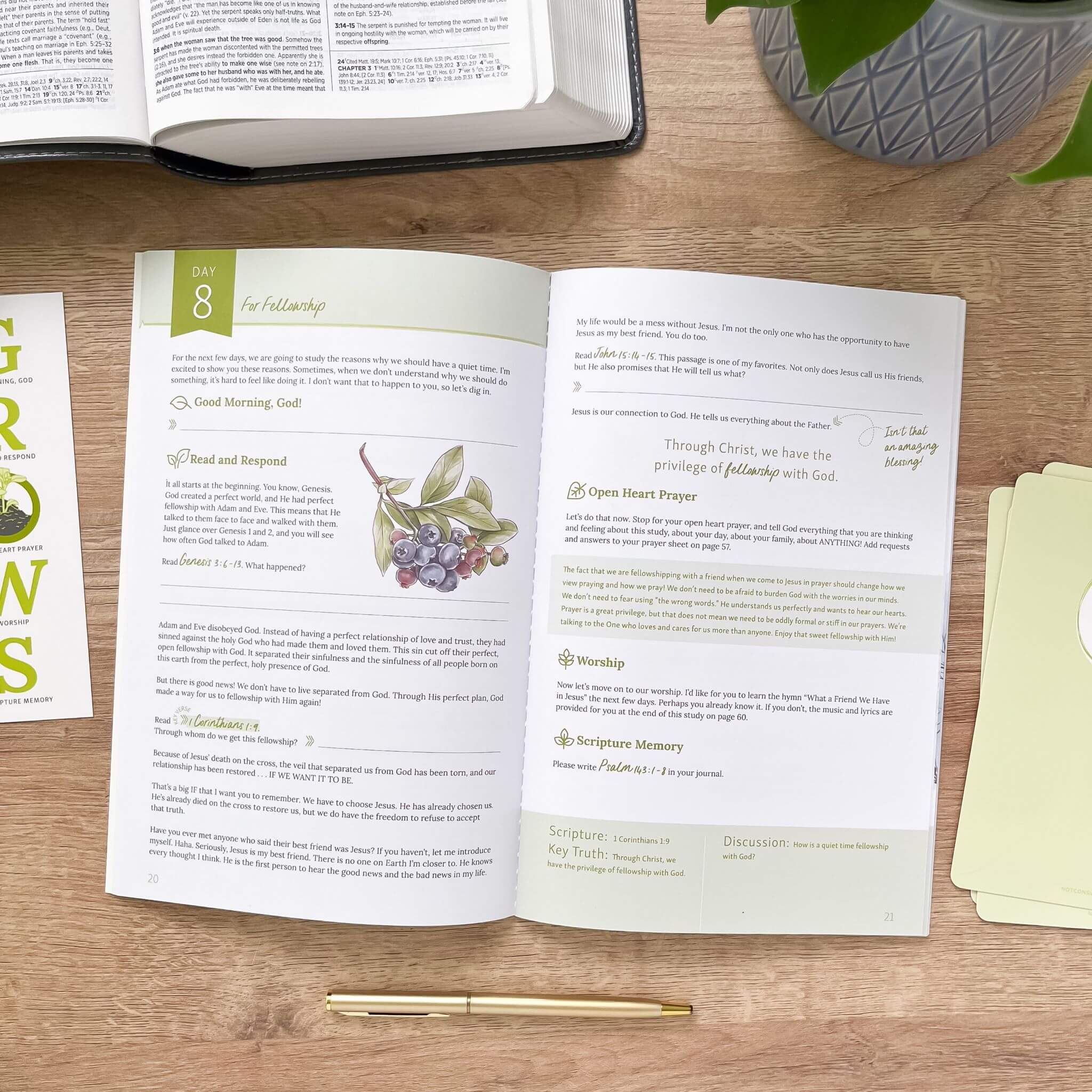The image depicts a neatly organized wooden desk with a light grain, set up for a study session. In the upper left corner, there is a partially visible black-covered book, likely a Bible. To the right of the Bible, a white workbook, prominently open to a page titled "Day 8 for Fellowship." This is highlighted in a green ribbon, with accompanying pale blue-green text reading "for Fellowship," decorative leaves, and headings like "Good Morning God," "Read and Respond," and a lengthy quote stating "Through Christ We Have the Privilege of Fellowship with God." Additional prompts include "Open Heart Prayer," "Worship," and "Scripture Memory," spread across both visible pages. Adjacent to the workbook on the left side is another artistic paper fragment displaying the partially visible word "grows." The upper right corner of the image showcases a potted plant with a diamond-patterned grey planter. Near the bottom of the image, a gold pen rests neatly beside a stack of rectangular cards positioned toward the lower right. Overall, the setting evokes a serene and organized atmosphere, ideal for religious study or reflection.